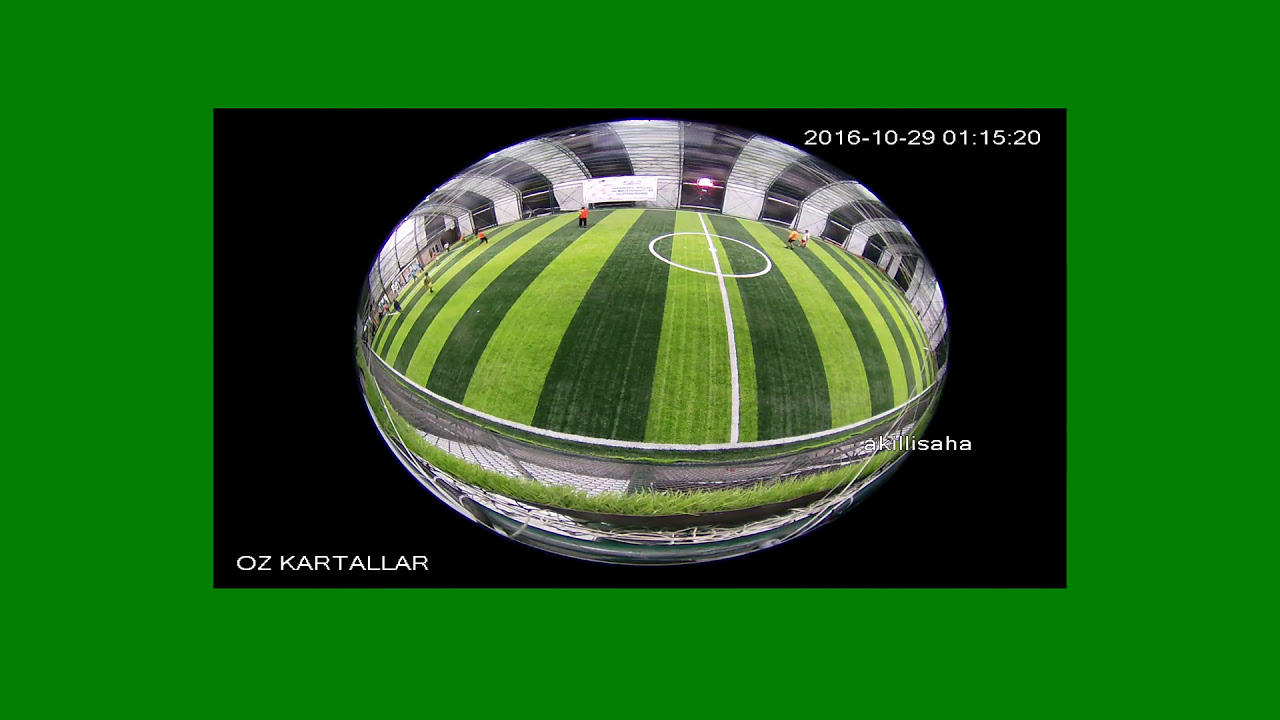The image is a detailed, panoramic view of an indoor soccer field. The scene is presented in an elliptical, fishbowl-like shape within a black rectangle, which is bordered by a green frame. The field itself is a mix of light and dark green, marked with white lines, including a central circle. Several players are visible on the field, notably wearing orange jerseys and black shorts, indicating active gameplay. The thick, solid black lines and interspersed windows in the dome structure add depth to the background.

In addition to the soccer action, the image contains several inscriptions. At the top right corner of the black rectangle, the date "October 29, 2016" and time "01:15:20" are clearly displayed, alongside a stamp mark with the name "Akilashit Saha," likely the artist's signature. At the bottom left corner, the name "Oz Carteller" is inscribed, which could refer to either the artist or a company. The vivid green and dark green hues of the grass contrast sharply with the black and white architectural elements, emphasizing the dynamic nature of the indoor soccer game.